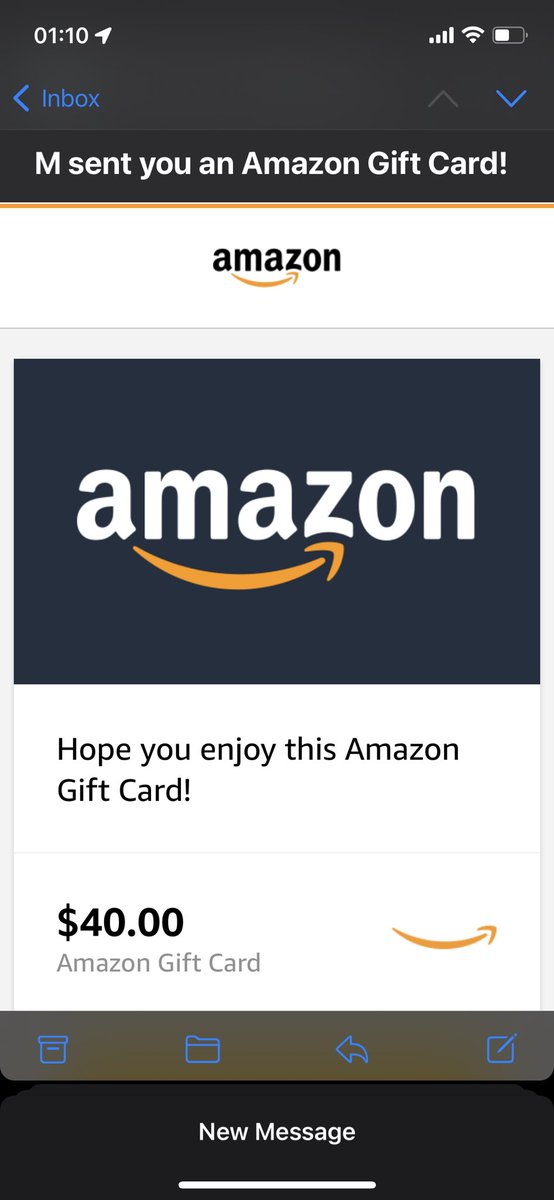The image displays a segmented user interface of a mobile device, specifically showcasing a messaging application. In the top left corner, the screen indicates '01:10', accompanied by an airplane mode icon, a four-bar Wi-Fi signal indicator, and a partially charged battery icon. Directly below this, on the left side, there is a blue-colored text that reads 'Inbox' next to a less-than symbol ('<'), suggesting a back navigation option. On the right side, a gray arrow pointing up and a blue arrow pointing down are visible, likely representing upload and download indicators.

Beneath this section, the interface has a black background with white text that states, "M sent you an Amazon gift card." Directly below this message, an orange line separates the content from a white background, which features the Amazon logo prominently displayed. Following this, there is a black rectangle containing another Amazon logo. Below this rectangle, a white area presents the text, "Hope you enjoy this Amazon gift card," along with a statement, "$40 Amazon gift card," denoting the value of the gift card.

The message thread is further divided by another orange line encompassing a curvy arrow marking. At the bottom of the display, the screen shows various icons typically found in a smartphone interface. Finally, there is a discernible 'New Message' prompt with a white line beneath it, suggesting the field where users can type a new message.